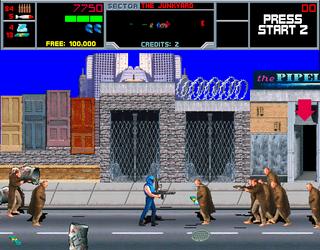This is a full-color screenshot from an unknown video game with primitive graphics. The background features a decrepit cityscape, highlighting a gray stone building topped with barbed wire and another adjacent structure labeled "P-I-P-E-L." A red arrow points downward into an open doorway in this building. Dominating the center of the image is a character clad in a blue helmet and blue uniform with exposed arms, wielding an assault rifle. This central figure is surrounded by numerous adversaries wearing long brown capes and brown pants, some of whom are armed. Behind the protagonist, more enemies in similar attire are advancing, one notably armed with a machine gun. At the top of the screen, the game's interface displays various details: the player's score of 7,750 points, two helmet icons indicating lives, a prompt for earning 100,000 points for free, two credits remaining, the current area titled "Sector: The Junkyard," and a "Press Start 2" instruction.